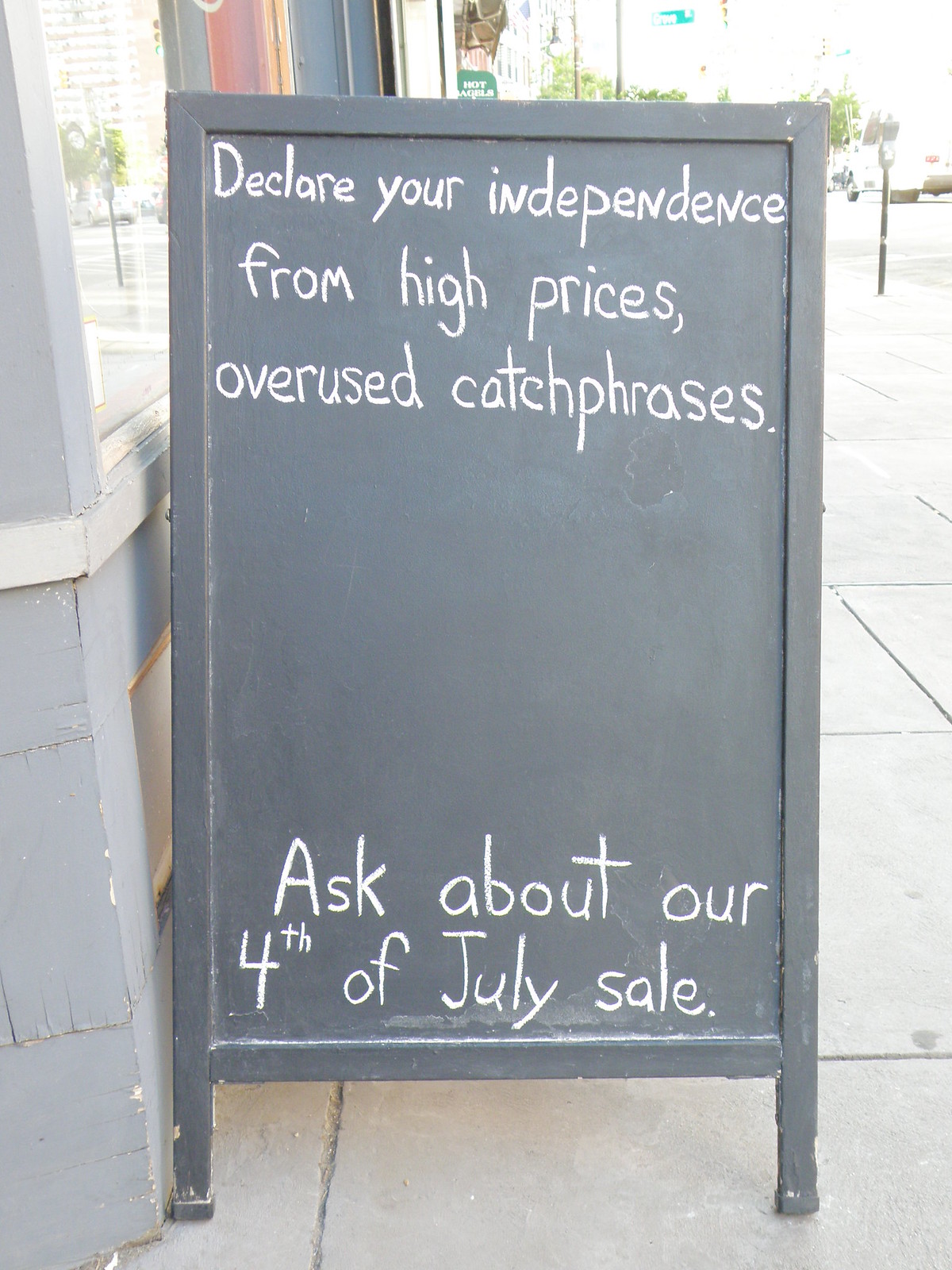In front of a storefront on a busy street, a gray-painted chalkboard sign prominently declares in white chalk, "Declare your independence from high prices, overused catchphrases." Beneath this, the sign encourages, "Ask about our 4th of July sale." The board, situated on a sidewalk, stands against a gray-painted stone building with a large glass window. Surrounding the area, you can see a bustling street with a parking meter, various vehicles, and a green street sign in the background. The environment features additional buildings painted in red, white, and blue, along with green awnings and trees lining the street, though the sign remains the clear focal point of the image.